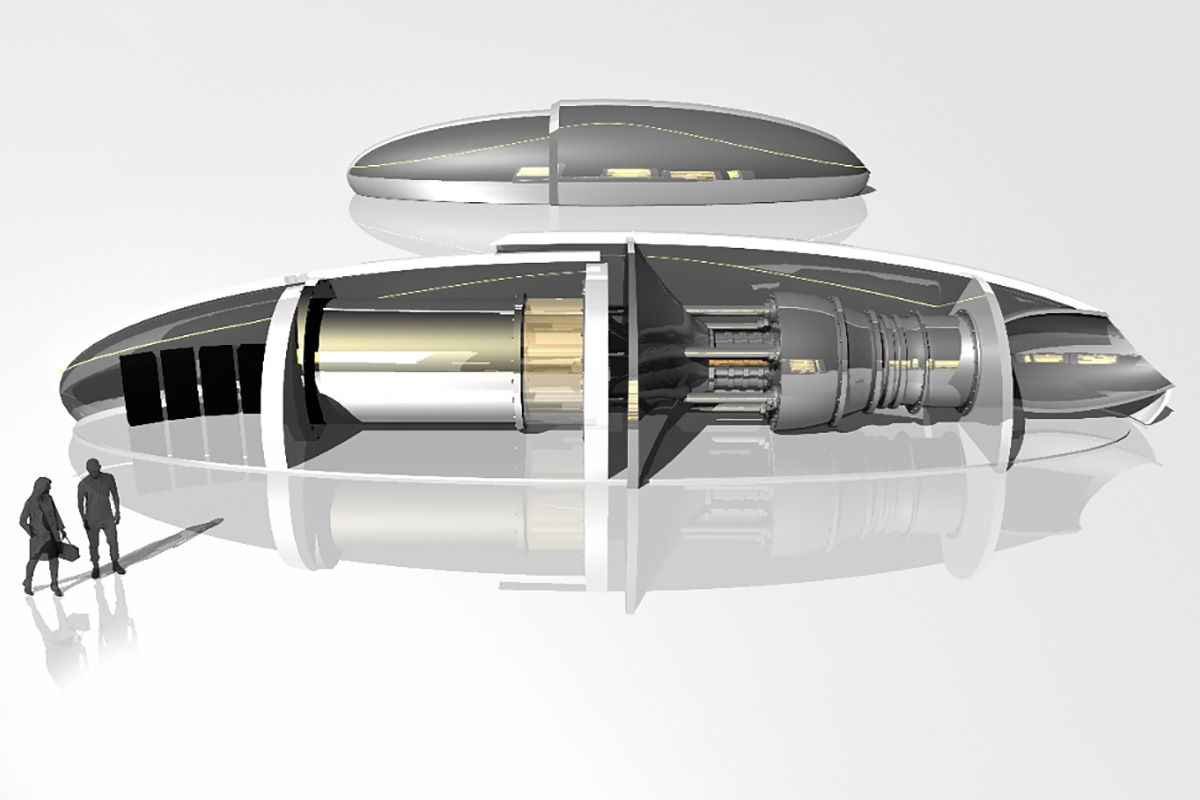This is a detailed 3D render of a futuristic tunnel system or cylindrical device set against a gray background. The device, featuring intricate machinery, includes four black boxes on the left and two inner cylinders. The top of the structure has a hovering lid-like element, while long strips of light illuminate the interior. In the foreground, two gray-silhouetted individuals—a woman with shoulder-length hair holding a duffel bag and a man in a t-shirt and jeans looking down—stand facing the device. They are positioned such that their reflections and shadows are clearly visible on the ground. An inset image above the device provides an external view, as though illustrating what the two individuals are observing. No text or labels are present to identify the purpose of this intriguing object.